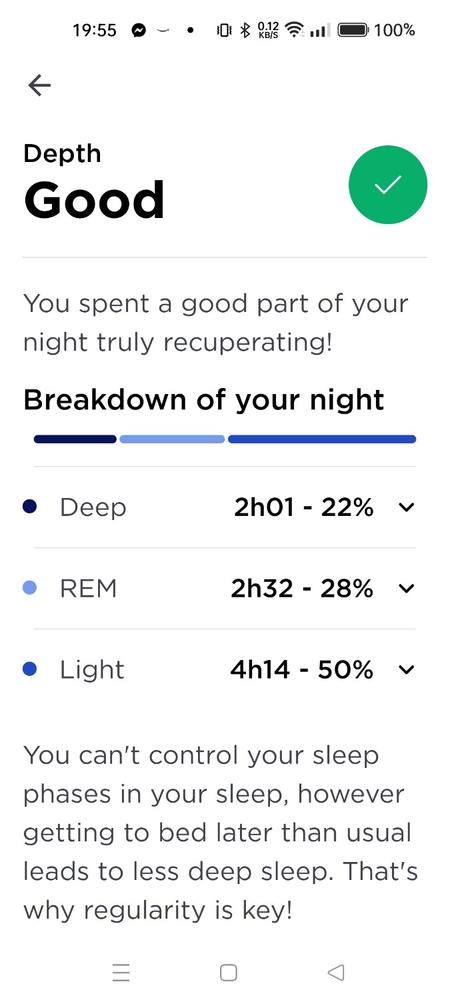A detailed screenshot from a mobile phone displaying sleep habits. The time at the top of the screen reads 19:55 (7:55 PM), five minutes before 8 in the evening. The user is currently active on the Messenger app, indicated by a smiley face icon in a small, circular dot. The phone is set to vibrate mode, with Bluetooth enabled, and shows a data transfer rate of 12 kilobytes per second. The Wi-Fi is connected with a signal strength of three bars, and the battery is fully charged at 100%.

Below these icons, there's a black, left-pointing arrow. Underneath this section, the text reads "Depth good" accompanied by a green circle with a white checkmark. The text further elaborates, stating: "You spend a good part of your night truly recuperating."

The breakdown of the sleep patterns is detailed with different shades of blue, specifying the duration and percentage of each sleep phase. The dark blue section represents "Deep" sleep, which is recorded as 2 hours and 1 minute, making up 22% of the night's sleep. This section has a dropdown arrow beside it. The light blue section indicates "REM" sleep, lasting 2 hours and 32 minutes, accounting for 28% of the sleep, also with a dropdown arrow. The royal blue section is labeled "Light" sleep, amounting to 4 hours and 14 minutes, or 50% of the total sleep, with a dropdown arrow.

A note below the breakdown advises: "You can't control your sleep phases in your sleep; however, getting to bed later than usual leads to less deep sleep. That's why regularity is key." Additional icons are displayed: three stacked lines, a clear square, and a clear triangle pointing to the left.